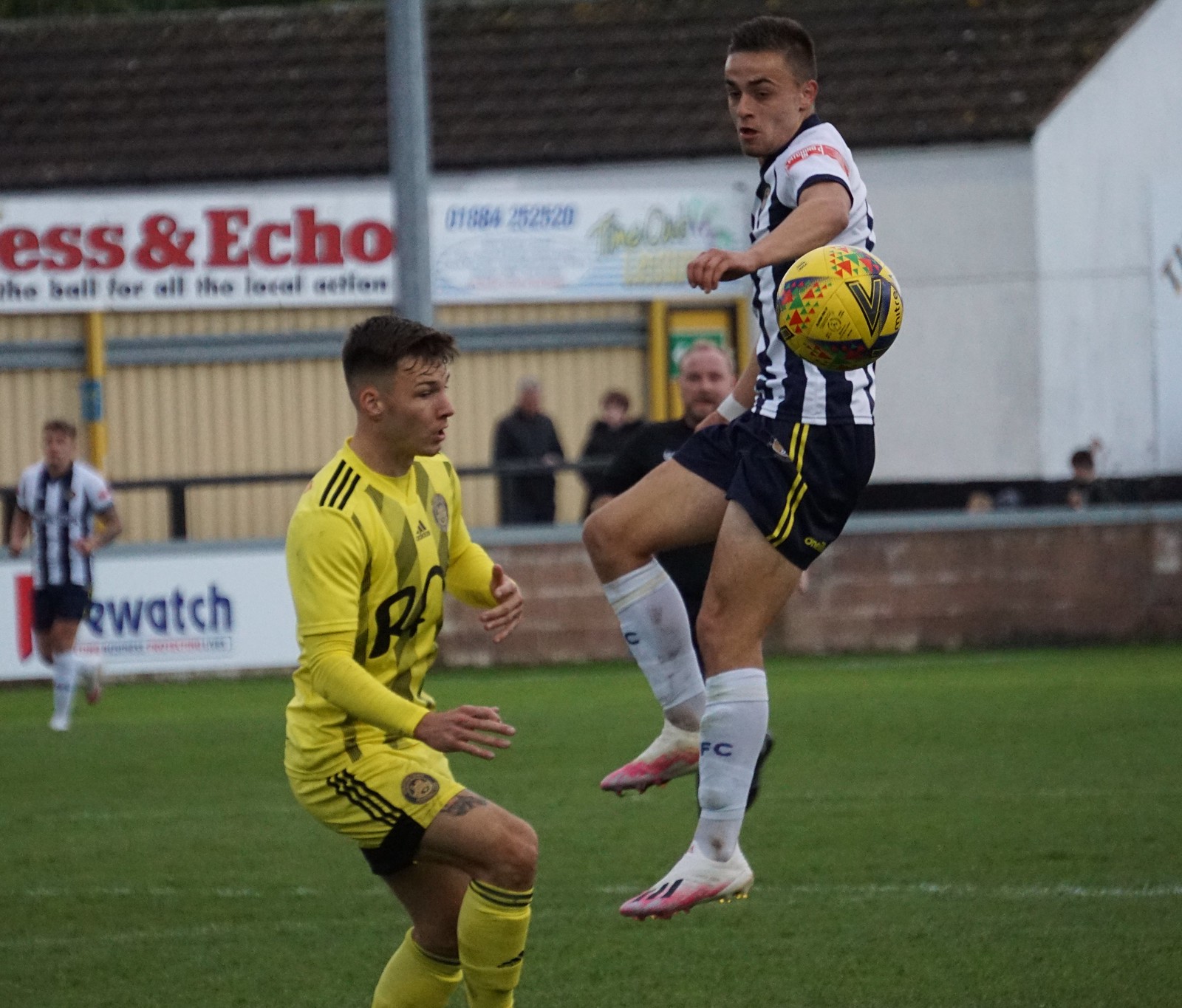In the image, two men are engaged in an intense soccer match on a lush green outdoor field. The player on the left, dressed in a yellow uniform with matching socks, shorts adorned with three black stripes, and a yellow jersey with black text, is positioned facing right and appears ready to make a move for the ball. His opponent, clad in black shorts with two yellow stripes, white socks, and a black and white vertically striped shirt, is captured midair, with his feet aligning with the yellow-uniformed player's knees, both focusing intently on the yellow-and-black soccer ball between them. Their hands are extended, emphasizing the dynamism of their play.

In the background stands a white building with a brown tiled roof, featuring a banner—possibly reading "B-Watch" or "Re-Watch." The building's courtyard is separated from the playing field by a waist-high wall, and several spectators, including a partially visible referee and another man in a black and white striped uniform, are observing the match. Among the scenery, a white line on the grass and a large metal bar are visible, and a basketball can be seen indoors behind the scene. The whole setting captures the vibrant and energetic atmosphere of the soccer game.